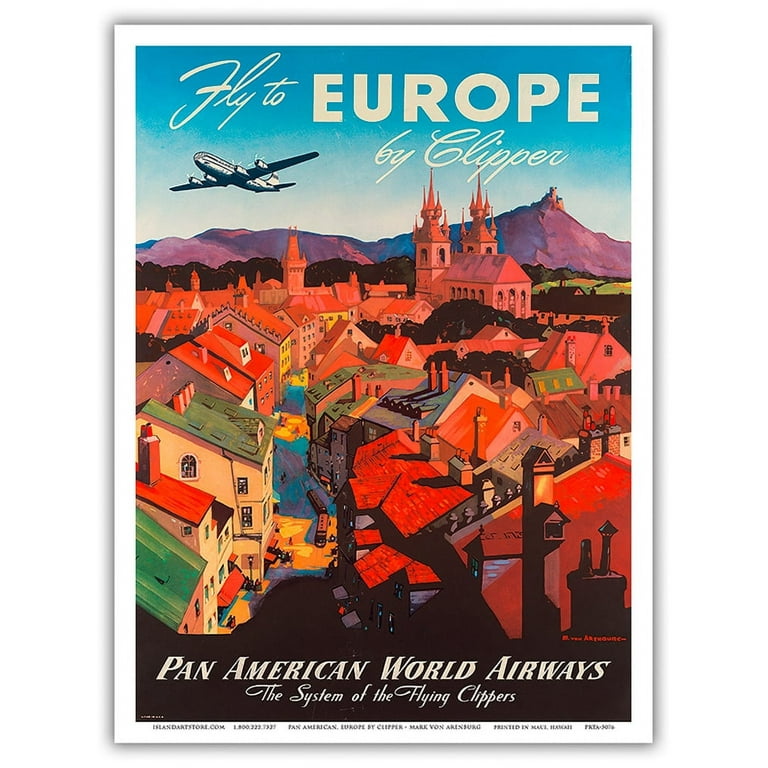The poster features a digitally crafted, vibrant depiction of a European village set against a scenic backdrop. At the top of the poster, bold white text reads "Fly to Europe by Clipper," set against a deep blue sky with a vintage four-propeller plane soaring overhead. Below the sky, a picturesque mountain range with hues of purple, blue, and dark shadows looms majestically. In the foreground, a charming village with narrow streets and colorful, angled-roof buildings is vividly presented. The buildings showcase a palette of greens, corals, yellows, oranges, and a variety of other pastel shades, including pink, tan, white, and reddish tones. Notably, the roofs are adorned in oranges and reds, complete with chimneys adding to the quaint appeal. Amidst the vibrant streets, which are painted in sections of yellow, green, purple, and orange, a small bus navigates through the town. The village also features a remarkable two-steeple church with Russian design elements, reaching up from the back of the cluster of buildings. At the bottom of the poster, a line of text declares "Pan American World Airways, the system of the flying Clippers," along with smaller, less legible text. The overall aesthetic captures the allure and nostalgia of classic European travel destinations.